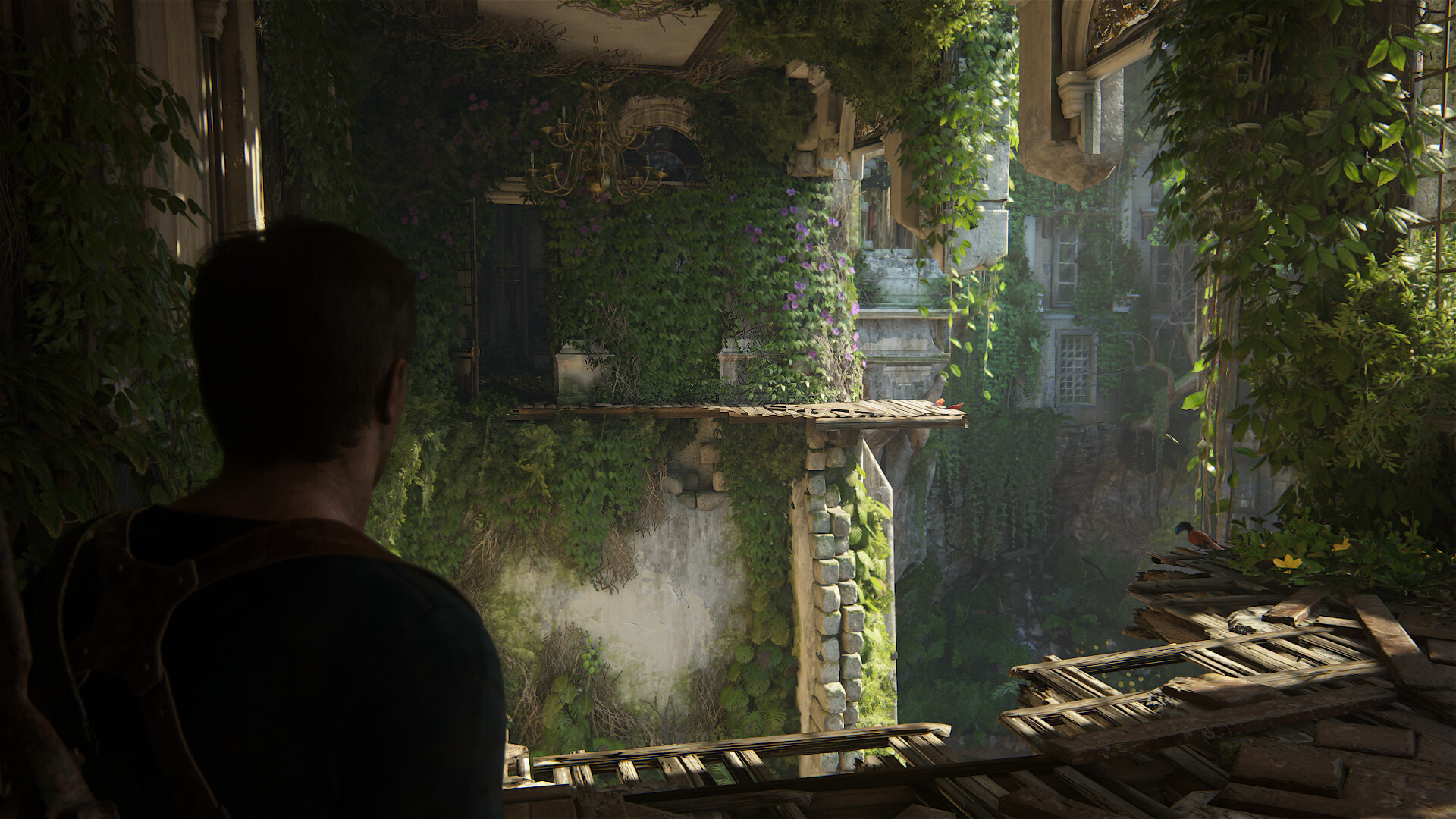In this detailed animated video game scene, we observe a character from the back on the left side of the image. The character, dressed in a dark gray shirt and brown vest, has short brown hair and is positioned slightly before a broken-off ledge. The ledge, appearing brown and deteriorated, lies to the character's right. Lush green leaves extend upwards towards the top right corner of the scene. On the left, the remains of a partially demolished building can be seen, with vibrant greenery infiltrating its structure. In the background, numerous building structures are visible, accented by an abundance of hanging green foliage, creating a sense of a post-apocalyptic, nature-reclaimed cityscape.